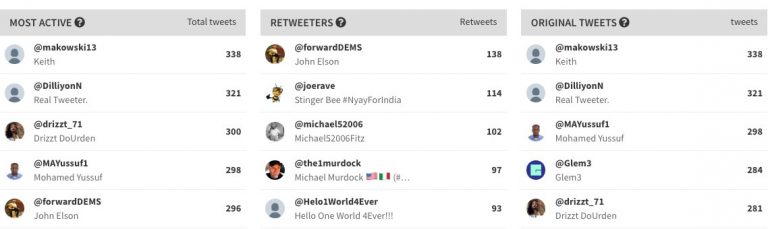A screenshot from Twitter’s analytics backend displays three distinct sections tracking engagement metrics for a user's account. 

- The left section, titled "Most Active Total Tweets," lists the top five users by activity. Each entry includes a Twitter profile picture, handle, and the total number of retweets they have achieved. 

- The center section, titled "Retweeters," showcases the top five users who have retweeted the account's content the most. Again, it includes profile pictures, handles, and the total retweets per user.

- The right section, titled "Original Tweets," identifies the top five users who have tagged the account in their original tweets. This section also presents profile images, handles, and the number of tweets each user has made.

Some Twitter handles displayed include recognizable names like Macowski13, DillianN, and Glemm3, alongside handles comprised of seemingly random letters and numbers, indicating a mix of active users interacting with the account. This analytics dashboard provides insights into user engagement, highlighting who is most actively engaging with the content.